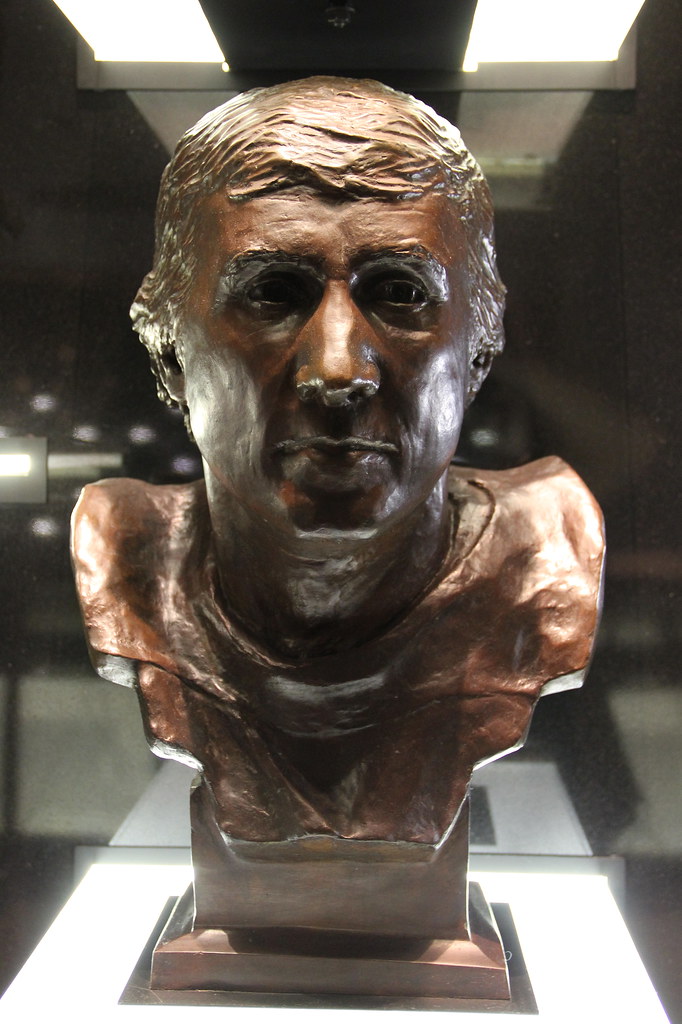This photograph, taken inside a museum, showcases a distinguished bronze bust of a man who appears to be Fran Tarkenton. The statue, composed of a lustrous brown metal that could be bronze or copper, intricately details the man's short hair and clean-shaven face. His facial expression is neutral with a closed mouth and eyes that gaze slightly to the right. The bust extends down into a rectangular base without any arms, capturing only the upper torso and shoulders. It rests on a metallic stand illuminated from below, housed within a clear glass case that features a locking mechanism. The case is further lit by two overhead lights, creating a display that accentuates the bust's features. In the background, ceiling lights run vertically, and a collection of white square lights is visible along the left, although the rest of the setting remains out of focus, drawing complete attention to the art piece.